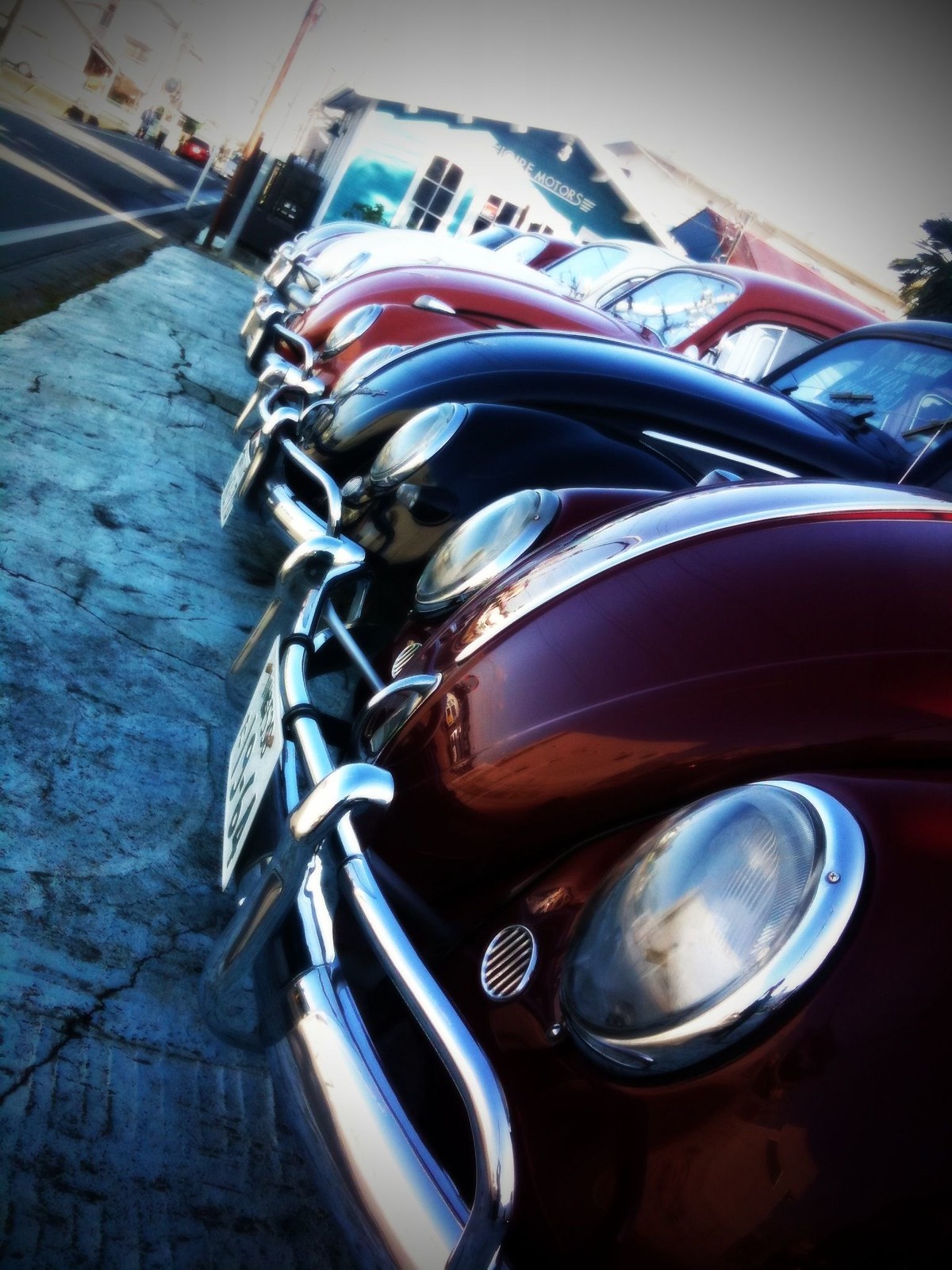The image captures a daytime outdoor scene at a car lot, probably belonging to a motor store, where five Volkswagen Beetles are neatly parked in a row. The lineup includes cars in various colors: white, gray, red, black, and burgundy. All the Beetles appear to be older models with chrome bumpers and circular headlights. The photograph is slightly tilted downwards and towards the left, creating a diagonal perspective where the street on the far left appears slanted. The cars are closely framed, showing primarily their front halves. There's a noticeable sun glare affecting one part of the image, causing some of the tile on the building's signage to be cut off, making it partially unreadable. Despite this, "motors" can be discerned from the building sign in the background. The overall condition of the cars is mint, and there's a license plate visible on the front of each vehicle.